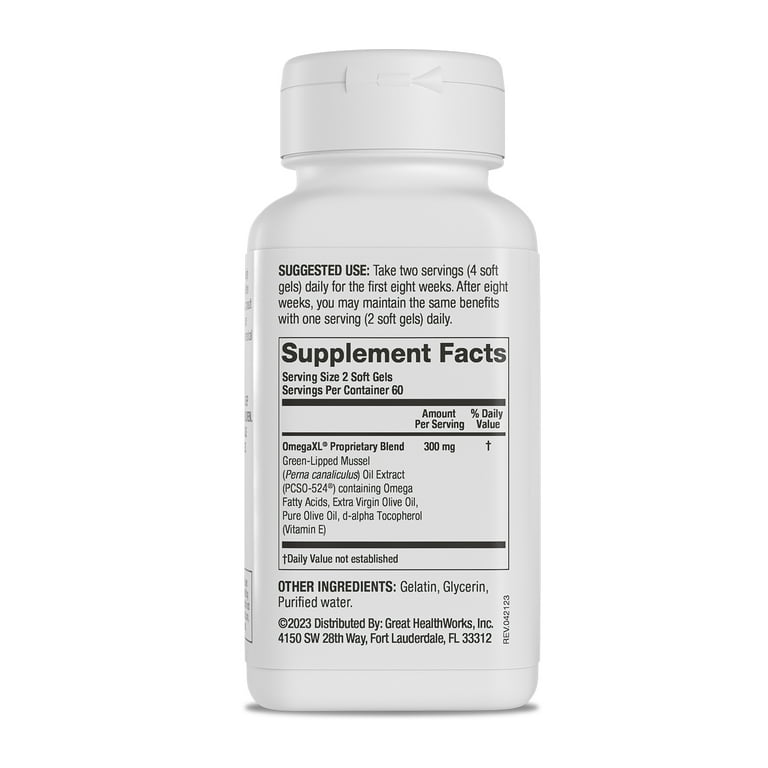The image depicts the back of a white plastic pill bottle with a cap that appears to be either a pop-off or screw-on type, currently screwed on. The label is white with black text. At the top, there is bold text indicating "Suggested Use," which instructs to take two servings, consisting of four soft gels, daily for the first eight weeks, and then maintain the benefits with one serving thereafter. Below this, there is a bold "Supplement Facts" box that provides details such as the serving size being two soft gels and servings per container totaling 60. It lists the contents, including 300 milligrams of Omega XL proprietary blend featuring Omega fatty acids and pure olive oil. The label also includes additional ingredients like gelatin, glycerin, and purified water. Towards the bottom, distribution information is provided, indicating the supplement is distributed by Great Health Works Inc., located at 4150 Southwest 28th Way, Fort Lauderdale, FL 33312, along with a 2023 copyright notice and a revision date of REV 042123.